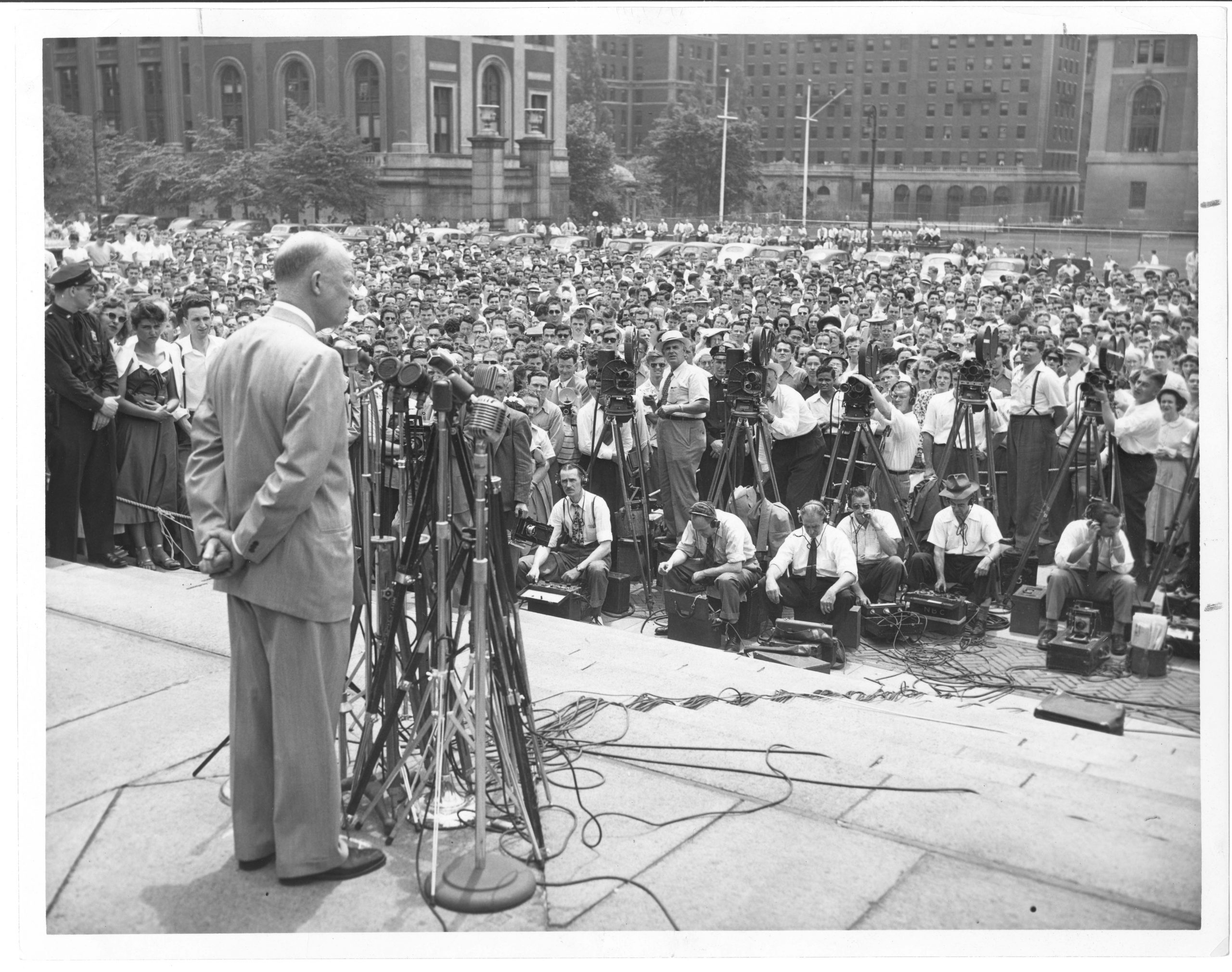A striking black-and-white vintage photograph captures a man in a suit, reminiscent of a scene from Forrest Gump, standing before an immense, bustling crowd in a downtown area. The man, hands clasped behind him, is surrounded by an array of at least 20 microphones connected to numerous amplifiers, while overhead daylight suggests the scene takes place at midday. Photographers, reporters, and video equipment fill the immediate vicinity, with five video cameras mounted on tripods prominently visible. Technicians, many wearing headphones and operating electronic gear from open boxes, monitor the amplifiers at the base of the stage. A police officer stands to the left, maintaining order as hundreds of onlookers, packed tightly together, intently listen to the man's speech. The image, likely from the 1950s or 1960s, evokes a sense of historic importance, capturing a moment of public address that drew a considerable, attentive audience.